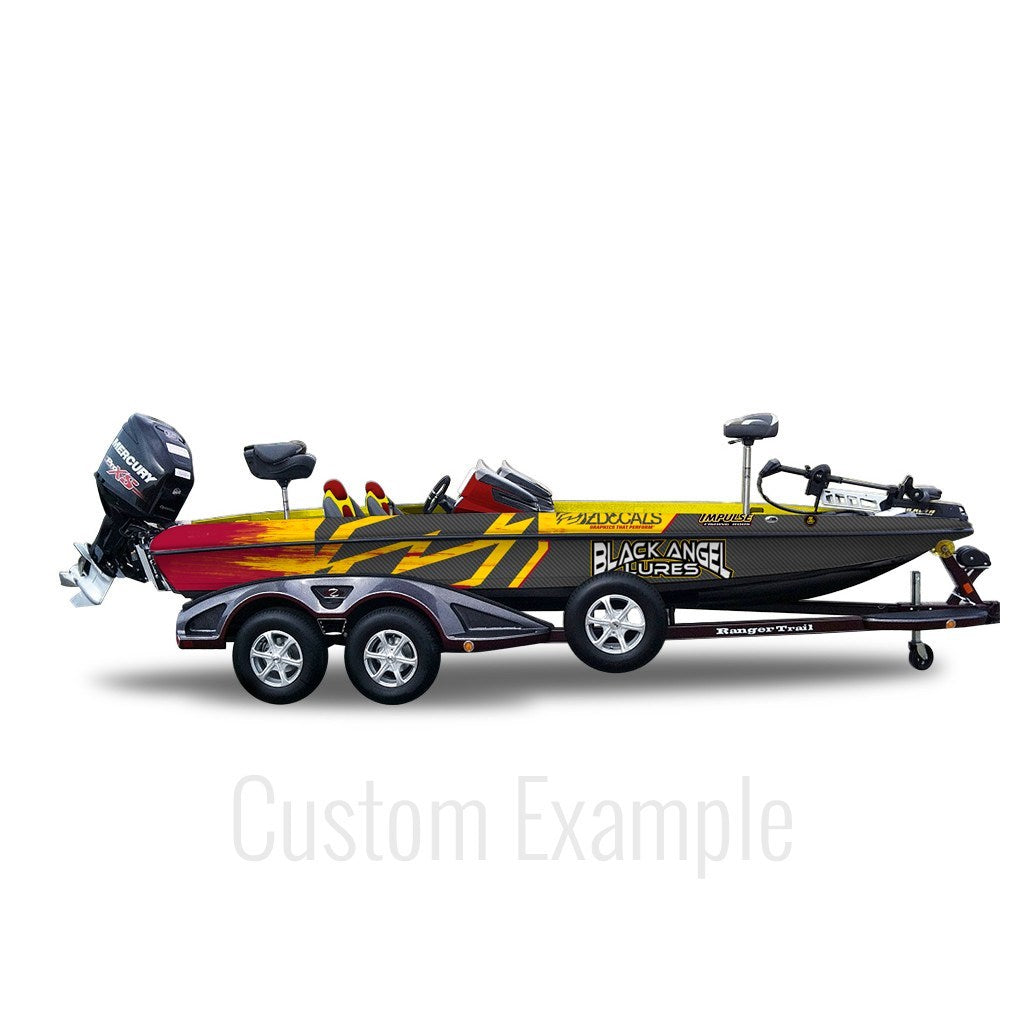This image is a side angle of a speedboat, which appears to be a digitally generated example. The speedboat is mounted on a black trailer, labeled "Ranger Trail," with a total of three wheels visible on the right side: two towards the rear and one located about midway with an additional small retractable wheel near the trailer hitch. The boat features a dynamic flame pattern that transitions from red to yellow near the back, indicating a fishing motif. The boat also displays various decals including "Black Angel Lures," "Impulse," and some Z-shaped designs. The engine mounted on the left side is branded "Mercury Pro XS." The boat’s seating includes two primary seats near the pilot's wheel and an elevated black chair at the back, which resembles a fishing chair. There might be an additional seat in the front. In the background, the entire image has a white overlay with the text "Custom Example" displayed prominently, suggesting customizable options for color schemes and branding.